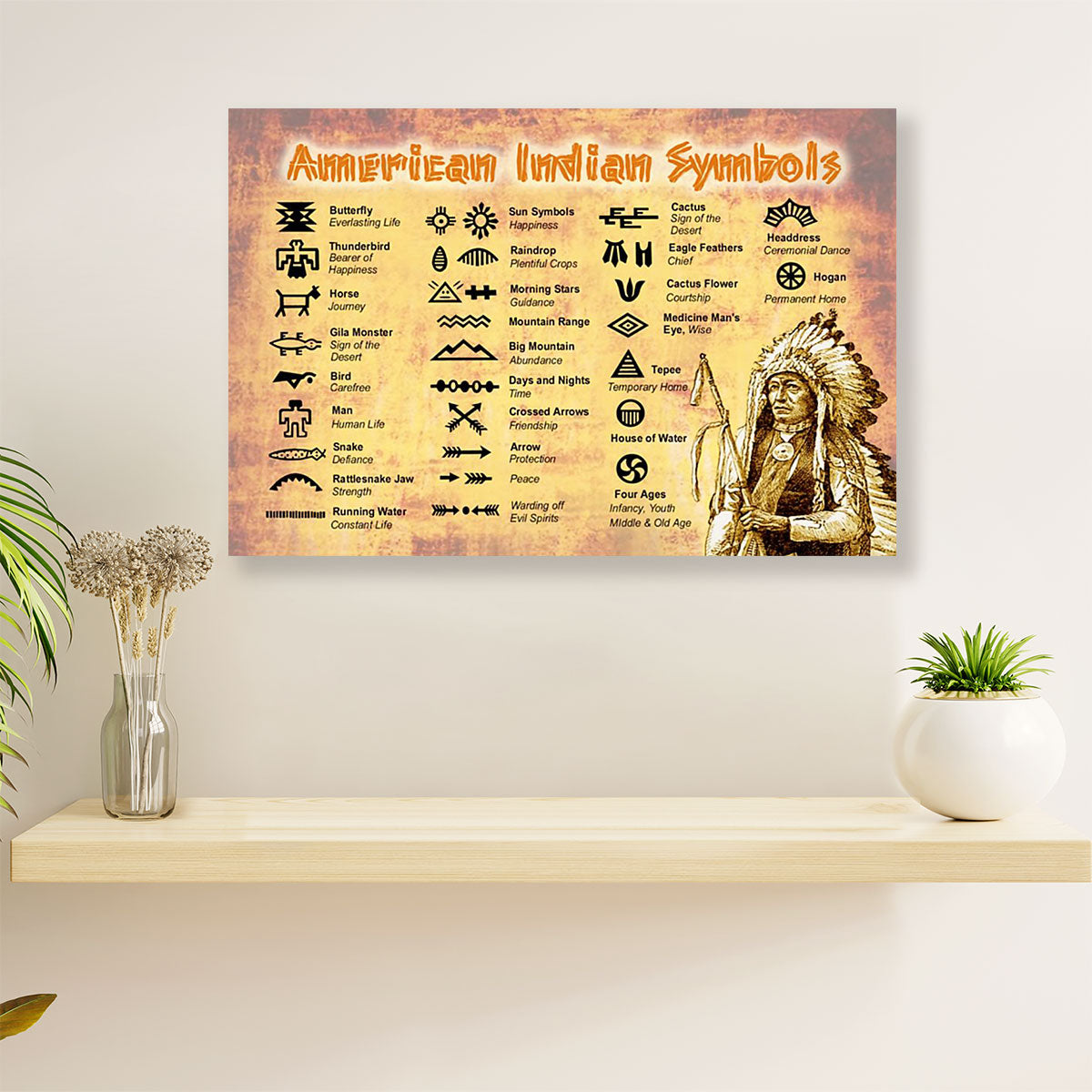The image depicts a living space with a white wall adorned by a floating light-wood shelf. On the left side of the shelf, there is a glass vase filled with light-colored, likely dried flower fluffs, presenting a slightly brown hue. To the right, in a white spherical pot, sits a small green leafy plant. A portion of another plant's green leaves can be seen peeking from the right edge of the image. The focal point above the shelf is a detailed poster titled "American Indian Symbols" in large orange text. This poster features a series of symbols commonly used in Native American culture, each with its name and meaning. Examples include the butterfly symbolizing everlasting life, the thunderbird as the bearer of happiness, and the horse representing a journey. The list also includes symbols for the gila monster, bird, man, snake, rattlesnake, running water, sun symbols, raindrop, morning stars, mountain range, big mountain, days, and nights, crossed arrows for friendship, and arrows for protection and peace, among many others. A prominent illustration of a Native American chief in full headdress and traditional attire is located in the lower right corner of the poster, holding a stick and looking towards the viewer. This illustration adds a rich cultural context to the otherwise contemporary interior design.